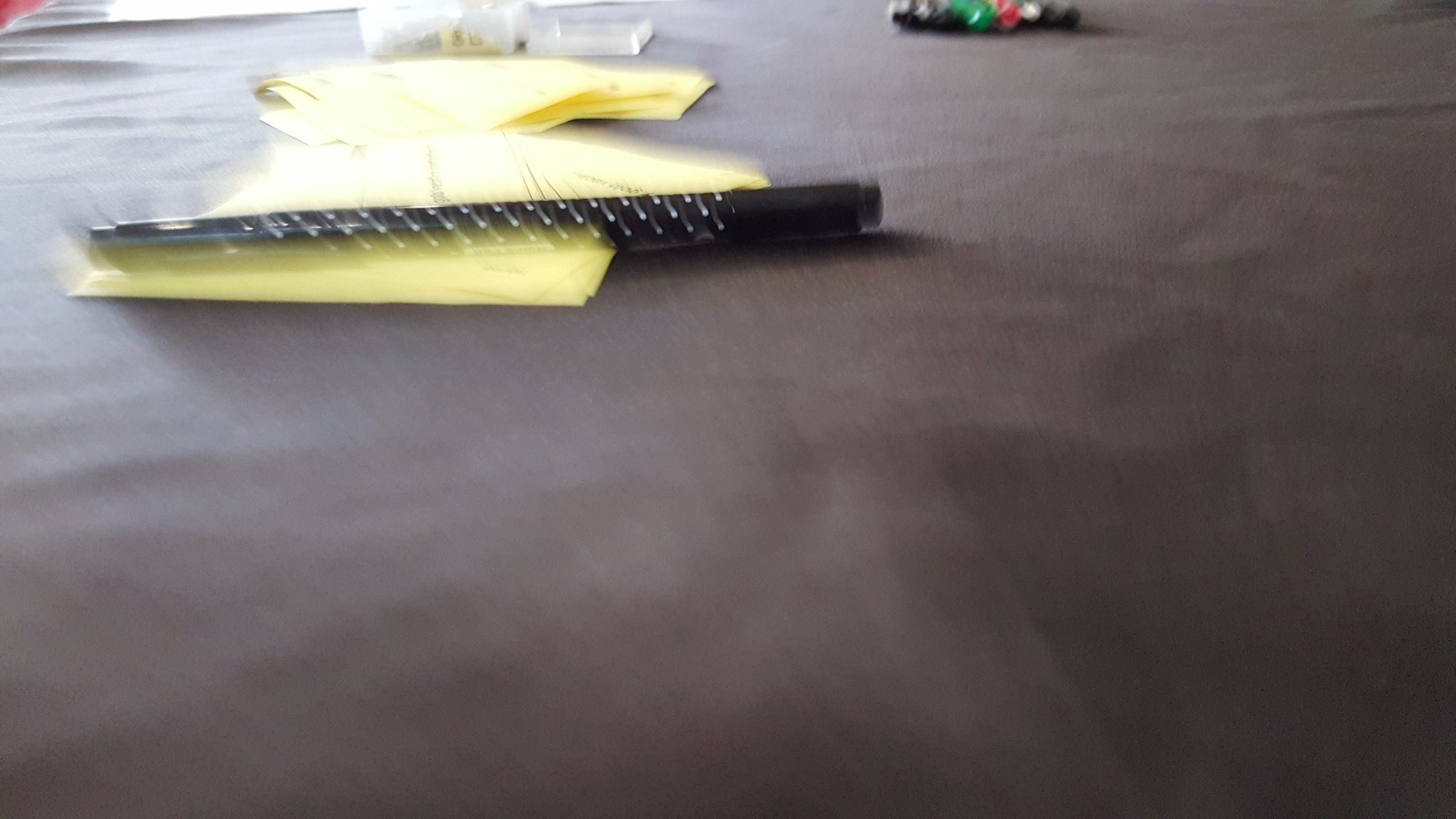This photograph shows a scene focused on a table, which appears to be either a pool or snooker table draped with a grey fabric covering. The material exhibits slight folds, adding texture and implying a soft, pliable fabric. In the upper left corner of the image, several yellow items that resemble sheets of paper are scattered. Additionally, a black object that potentially could be a pen lies horizontally across the table cover. Towards the top right of the image, a collection of colored objects that seem to resemble dice is visible, though details are blurred, making precise identification challenging. Overall, while the image is slightly unclear, the arrangement of objects suggests a casual or preparatory setting.